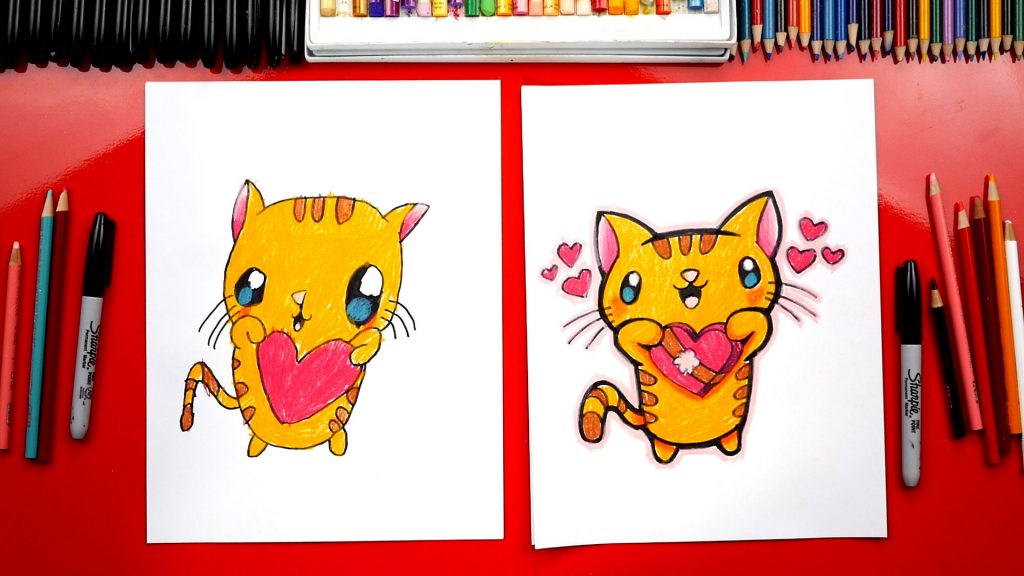This detailed image captures a top-down view of an art setup on a shiny red table, featuring an assortment of art supplies meticulously arranged around two central drawings. The supplies include black Sharpie markers placed on either side of the drawings, several colored pencils spread across the left and right sides, and various markers and pastels positioned at the top of the table.

The center of the composition showcases two white sheets of paper, each bearing a drawing of a cartoon-style yellow and orange-striped cat. Both cats share similar adorable features: blue eyes with black pupils that include a blue dot and white highlight, pink ears, a pink nose, open mouths revealing pink tongues, and three whiskers on either side of their faces.

The cat on the left appears to be an amateur drawing, possibly by a child, while the cat on the right is professionally rendered, suggesting it was made by a more experienced artist. Both cats display three stripes on their heads, bodies, and tails and hold pink hearts. The cat on the left grasps a heart up to its chest, whereas the cat on the right holds a heart adorned with a ribbon. Surrounding the head of the cat on the right are three small floating hearts on each side, enhancing the charm of the illustration. The background setup implies this might be a cozy art studio or a home crafting space, emphasizing the contrast between the drawings and creating a vibrant, creative atmosphere.